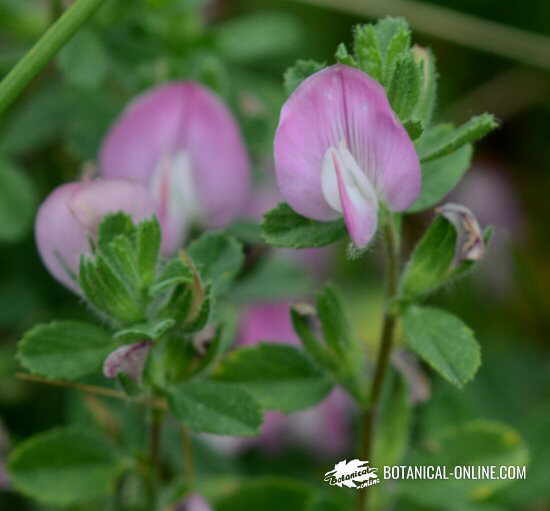This close-up image captures a collection of wildflower plants with short stalks and broad green leaves. The stalks are a darker shade of green, supporting several flowers characterized by petals of light purple to dark pink hues, with traces of white. The photograph prominently features two flowers in the foreground—one on the right and another on the left—that are in sharp focus, showing vivid purple petals. In the background, additional purple flowers and green leaves appear blurred. A darker green stalk runs diagonally across the top left corner. In the bottom right corner, the website "botanicalonline.com" is inscribed in white ink, accompanied by the site's leaf-shaped logo.